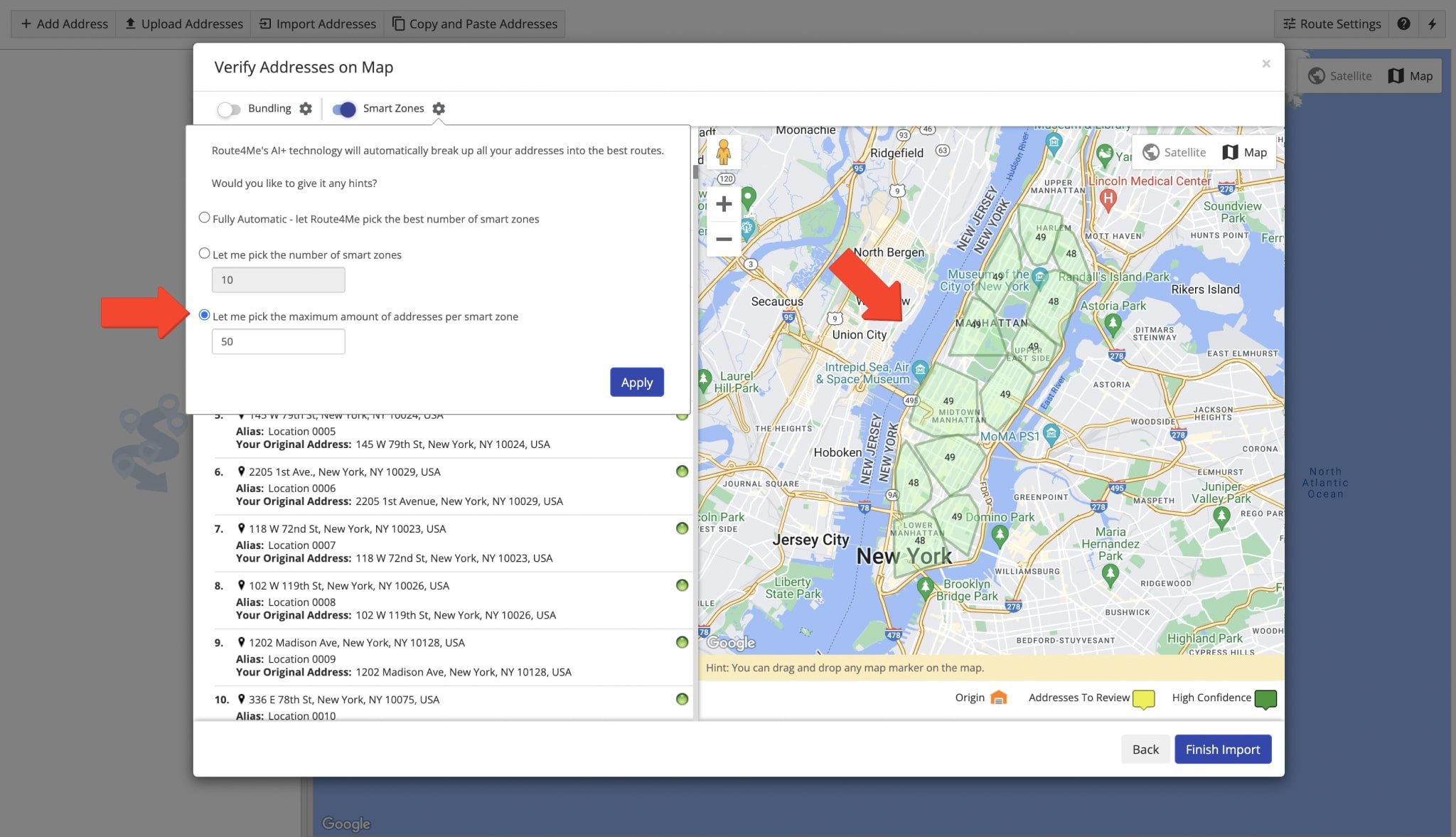The image, taken from a website, features a detailed map of New York, with various waterways prominently displayed. A thick red arrow points directly to the Hudson River, highlighting its location. On the right side of the screen, another large red arrow directs attention to a section of the website featuring an application tool. This tool is designed to optimize routes for multi-address trips using AI and technology. 

The tool interface includes several options for customization:
- A top section labeled, "Would you like to give it any hints?," which remains unselected.
- Three specific configuration choices:
    1. "Fully Automatic" (not selected).
    2. "Let me pick the number of smart zones," with a preset of 10 (not selected).
    3. "Let me pick the maximum amount of addresses per smart zone," with a preset of 50 (selected).

The red arrow is pointing precisely to the "Let me pick the maximum amount of addresses per smart zone" option, which has been clicked.